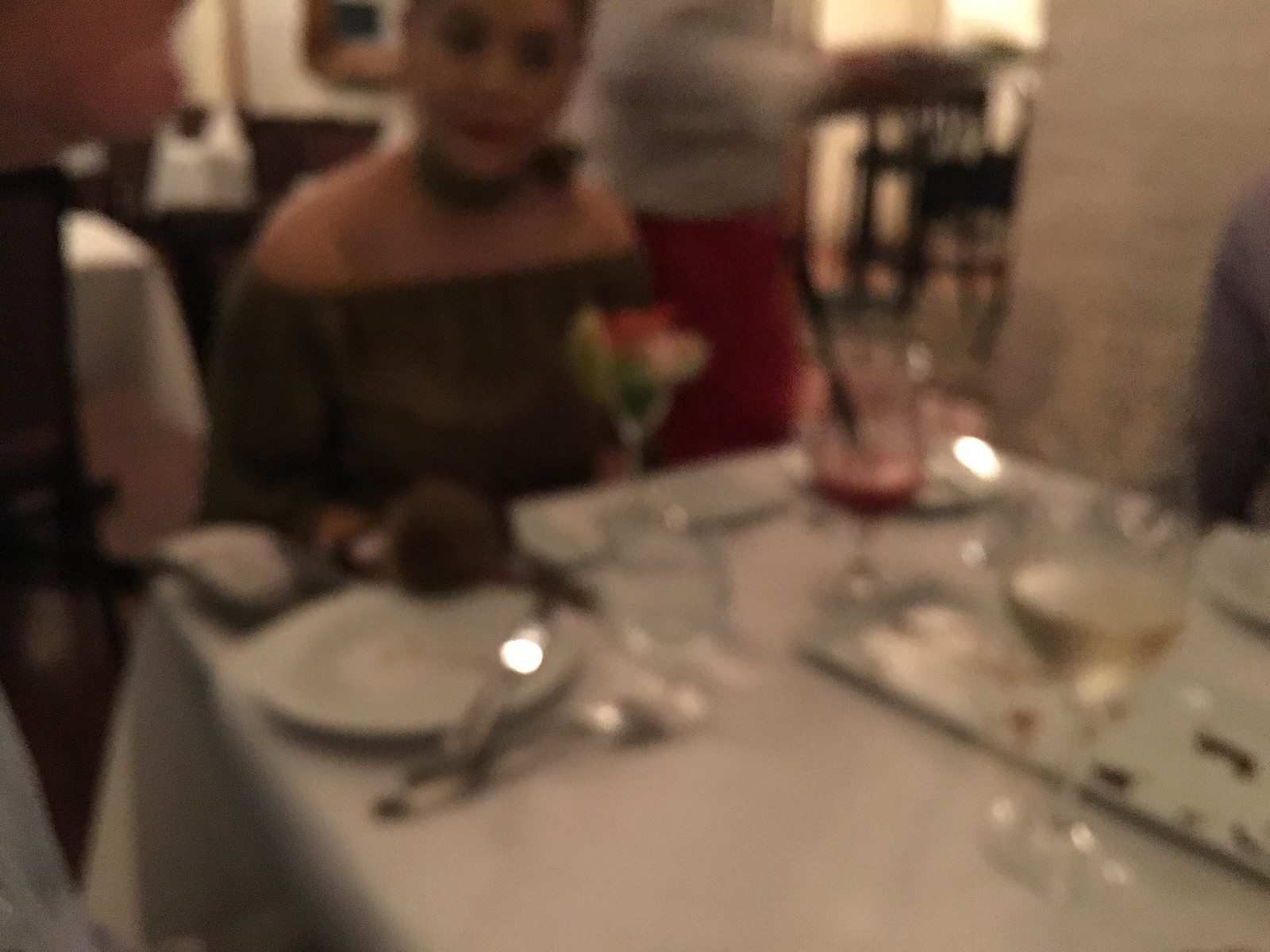In a dimly lit restaurant, a blurry, low-quality photograph captures a dinner table draped with a white tablecloth, set with used plates, silverware, and both a glass of red and white wine. The table is surrounded by at least three partially visible individuals, with one person on the right side only identifiable by their gray sleeve. At the head of the table sits a woman with a darker complexion, wearing an off-the-shoulder, two-tone blouse, and a green scarf or kerchief tied in a bow around her neck. The blouse exposes her shoulders up to her neck. In front of her is a cocktail glass, possibly containing a mixed drink or shrimp cocktail, adorned with a decorative paper umbrella or flowers. To her left, another individual, partly visible, appears to be wearing a light gray shirt. The surrounding scene features dark-colored chairs and other tables with similar white tablecloths, illuminated by overhead lights reflected in the glassware.